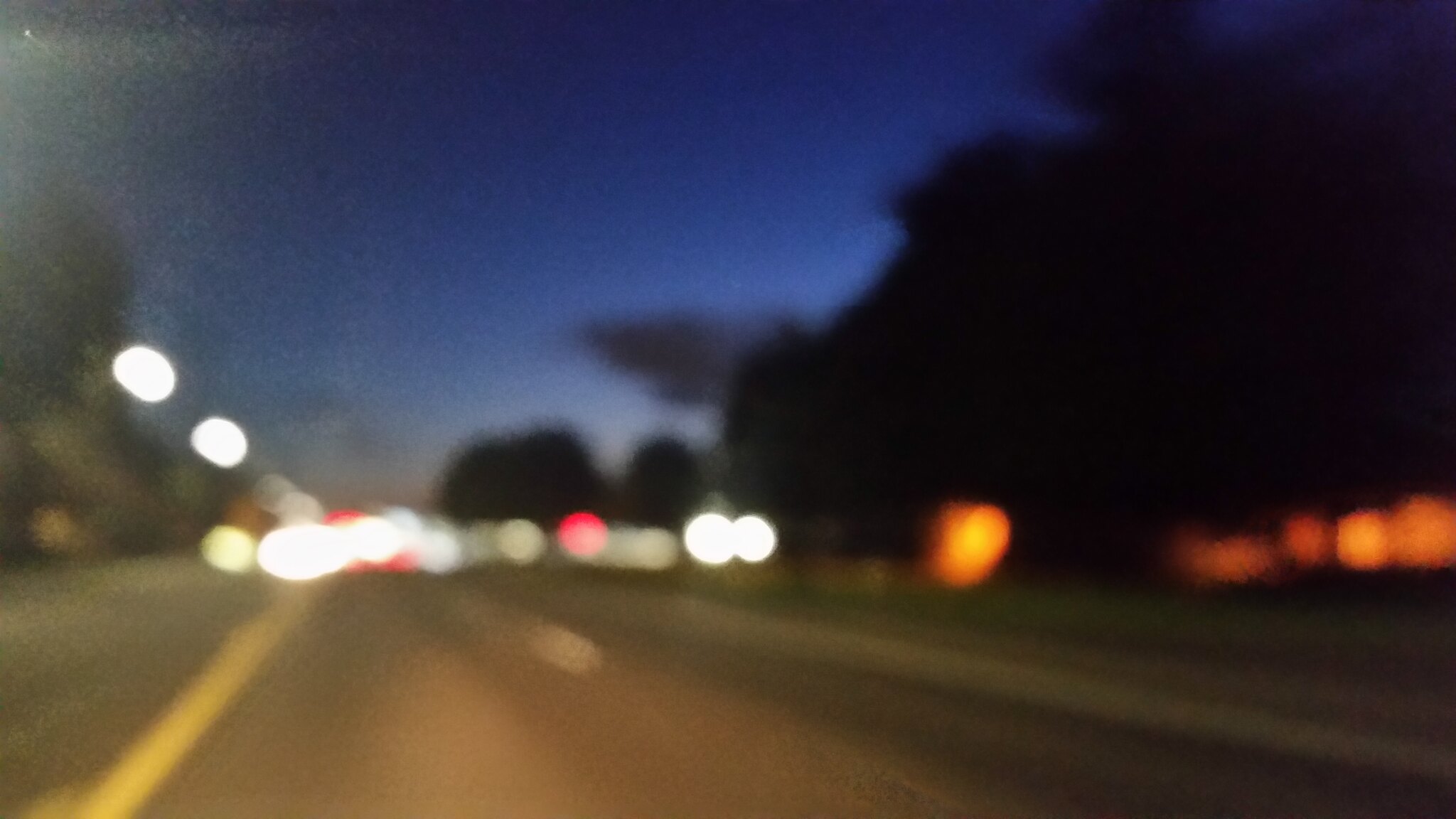A blurry nighttime photograph captures a roadway, likely taken from within a moving vehicle positioned in the left lane. The image showcases the contrasting white lane divider on the road, delineating the path ahead. To the left, a yellow divider line demarcates opposing traffic directions. The distant glow of car headlights pierces through the evening sky, now veiled in the deep hues of night. Silhouetted trees stand starkly against the darkened sky on the right-hand side, adding a somber, natural element to the scene.